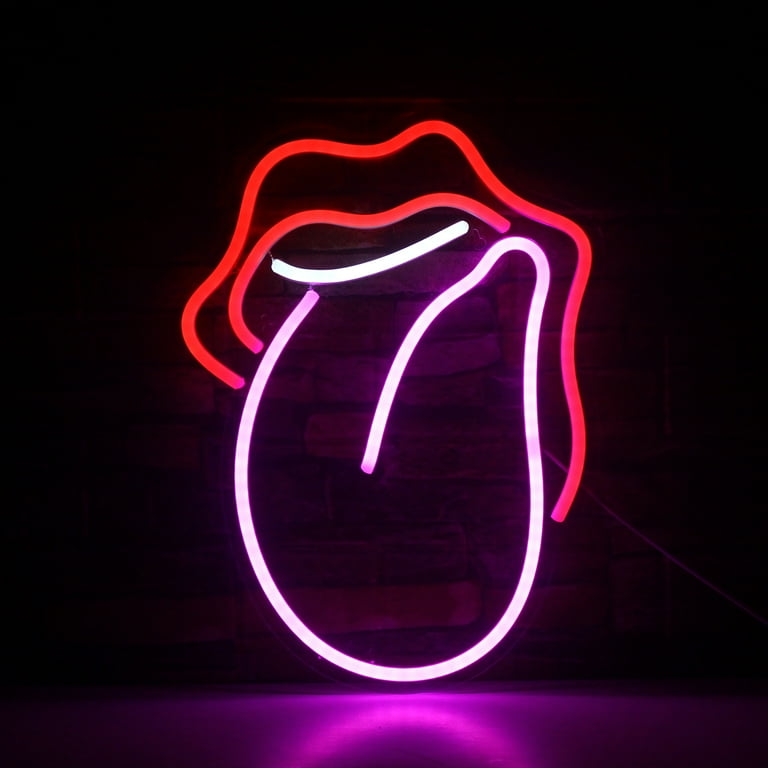The photograph depicts a neon sign in the center of the image, which is set against a brick wall in a dark room. The neon sign is designed to resemble the iconic Rolling Stones logo, featuring a pair of red lips with a light pink tongue sticking out. The lips have a bright red outline, while the tongue adds a light pink hue. Below the tongue, a purple glow illuminates the surface beneath, creating an intriguing effect. The brick wall serves as the backdrop, and an electrical cord extends from the right side of the neon sign, trailing downward. At the bottom of the image, there is a rectangular shelf that also appears to glow purple due to the neon light. The photograph is taken vertically, slightly taller than it is wide, and captures the neon sign effectively lit up in the dark, showcasing its vibrant colors and the detailed texture of the brick wall behind it.